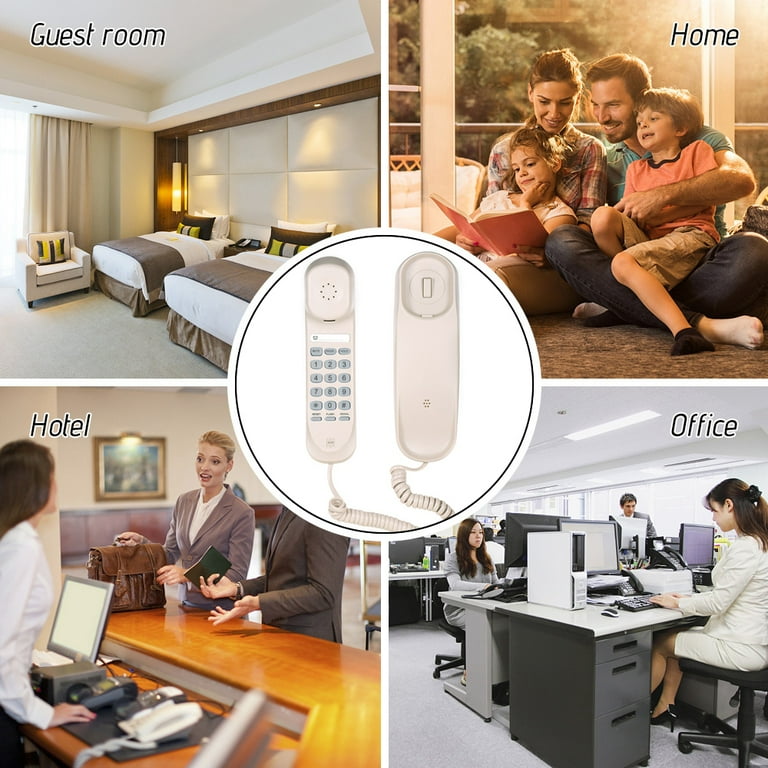This image is a composite graphic featuring four distinct scenes arranged around a central circle. In the middle circle, there is an old-fashioned touch-tone phone with a cord, reminiscent of the 80s and 90s. The upper left quadrant is labeled "Guest Room" and depicts a motel room with two double beds, white paneling, brown trim, and various pillows in brown, white, yellow, and blue. A small white chair and white curtains complete the room's decor. The upper right corner, labeled "Home," shows a family scene with a man and a woman each holding a child on their laps, reading a red book together. The bottom left section, titled "Hotel," illustrates a hotel reception area where a clerk in a white shirt assists two business people in suits, one of whom is carrying a briefcase. Lastly, the bottom right part labeled "Office" features several desks with men and women working on computers in a typical office environment. Each scene circles back to the central image of the classic corded phone, connecting the various settings through this nostalgic piece of technology.